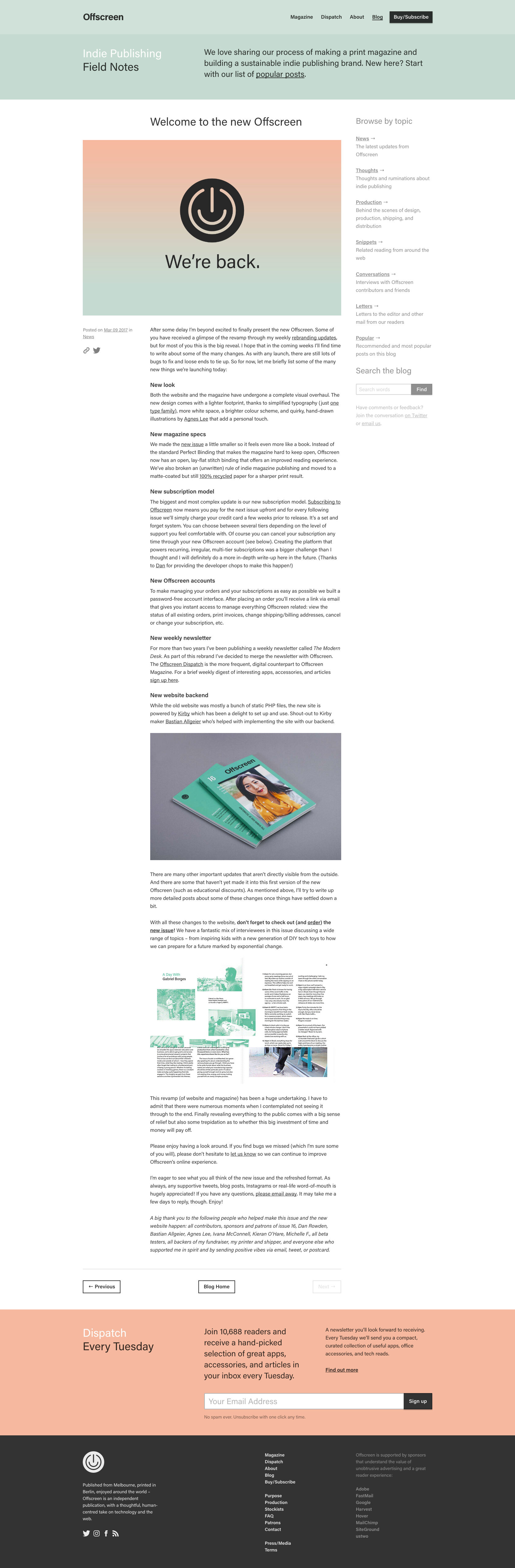This image is a website screenshot with visually dense content. At the top, there is a light blue border about an inch thick. Approximately an inch from the left edge, the word "Offscreen" appears in black, followed below by "India Publishing" in white, and then "Filled Notes" in black. Near the top-right corner, about an inch from the right side, there's a black tab with the text "Buy/Subscribe" in white. Next to this, "Blog" is underlined and written in black, followed by "Dispatch Magazine" also in black.

Just below "India Publishing", there are three lines of information pertaining to the website. The larger section of the page has a white background with the text "Welcome to the new Offscreen" prominently displayed in black at the center. Midway down, there's a pinkish rectangle with a light blue center featuring a black circle with an almost complete white line around it, and a smiley face within the circle. Underneath this graphic, the text "We're Back." is written in black. To the right of the graphic, it says "Browse Topic" and presents seven dropdown tabs, followed by a "Search the Blog" section with a search bar beneath it.

Continuing down the page, there are approximately seven paragraphs of information, followed by another image with a purple background and green, playing-card-like elements positioned diagonally from the top left to the bottom right. Below this image, there are two more paragraphs and a selection of small picture icons. The content then includes four additional paragraphs, ending with a two-inch pink border followed by a black border filled with an extensive amount of text.